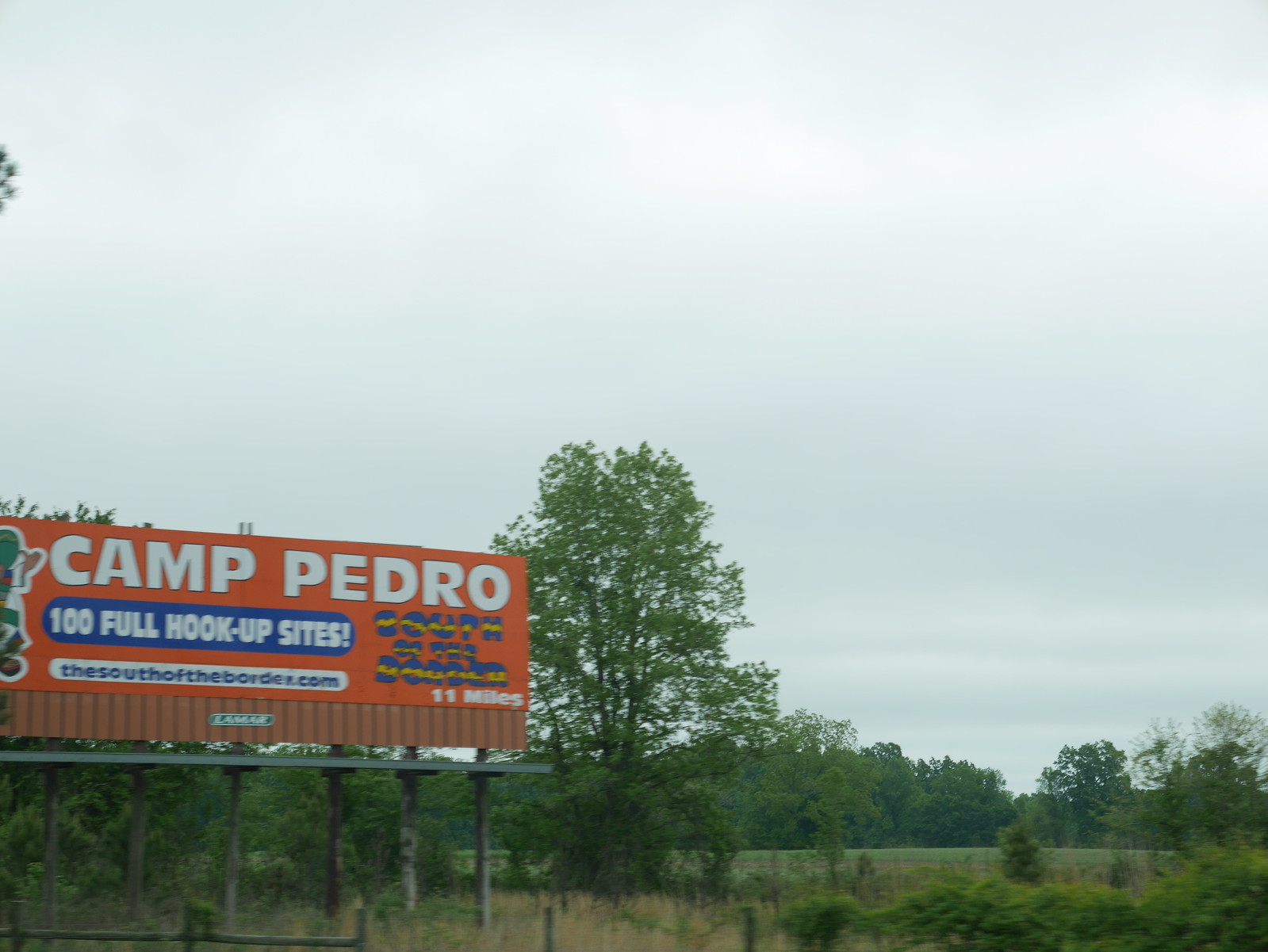This outdoor photograph captures a moody, overcast day with a dominant gray sky that covers approximately two-thirds of the image. Below the sky, a verdant green field stretches across the frame, sporadically dotted with a few trees and plants. The primary focus of the photograph is on the left side, where a prominent billboard stands tall, supported by multiple metal poles. The billboard is strikingly red, with bold white text that reads “Camp Pedro.” Below this, a blue rectangular bar features the message “100 Full Hookup Sites” in white font. Further down, the text “TheSouthoftheBorder.com” is displayed, followed by another line beneath "Pedro" that reads “South of the Border” in blue and red, with a directional note indicating “11 miles.”